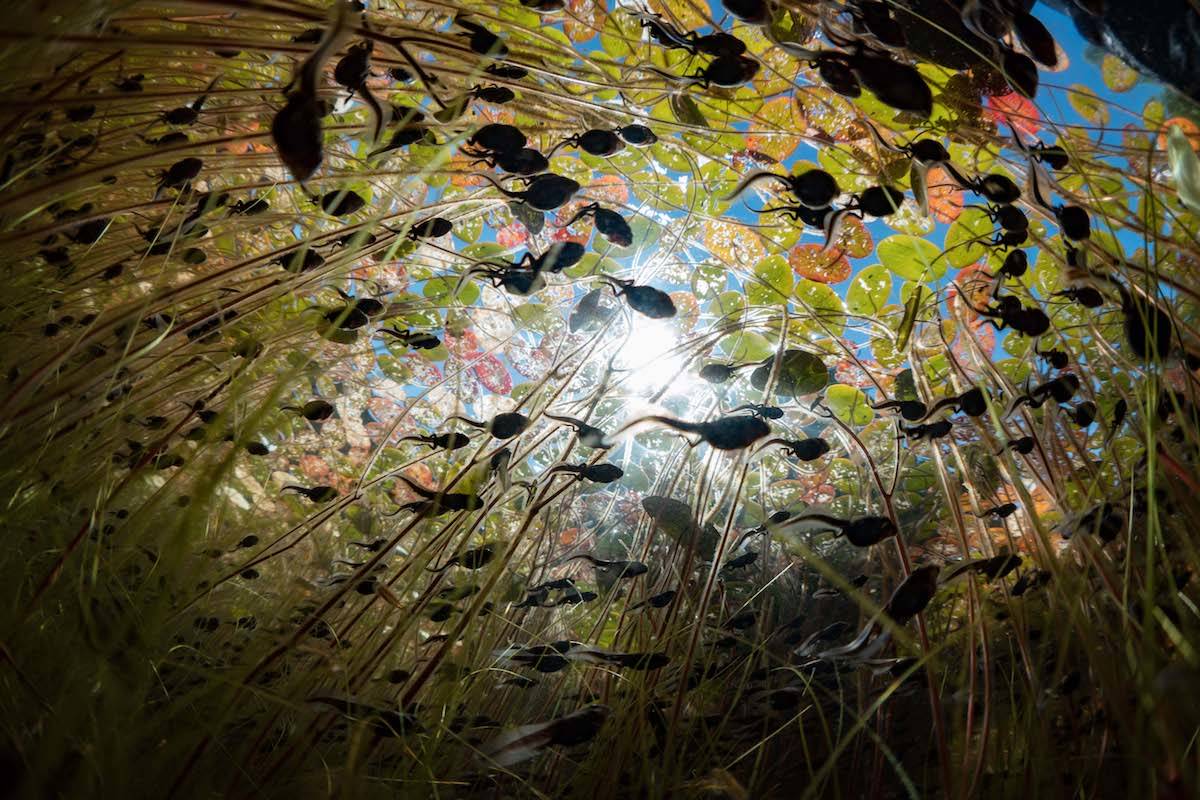The image captures an underwater scene with a view looking upwards in a pond. The photo shows a large cluster of tadpoles, or poliwogs, swimming around, many of them in varying stages of transformation into frogs. Some tadpoles already have legs while others are still more fish-like. They are dark black, with some bearing shades of black. Around them, lily pads float on the water's surface, with their roots extending downward into the water. The lily pads vary in color, some green and some red. Beyond the lily pads, the bright blue sky and a glowing, whitish sun can be seen, with rays streaming through the water towards the viewer. There's also a small fish swimming among the tadpoles, adding to the dynamic underwater ecosystem captured in the photograph.